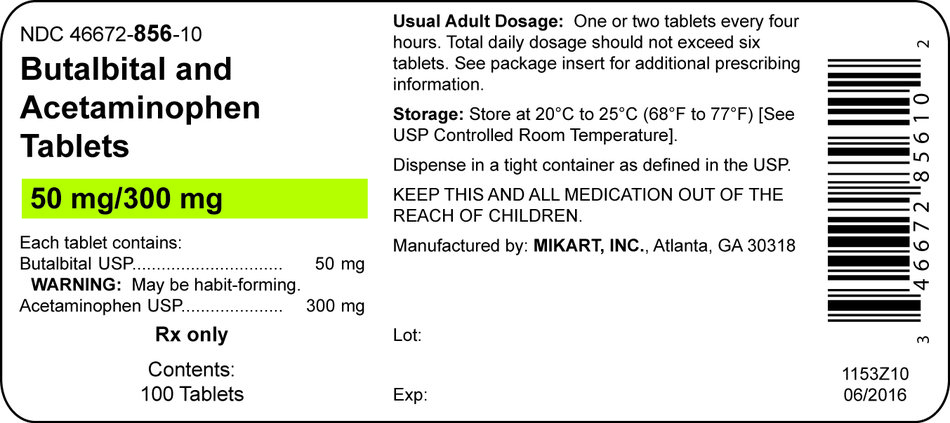Screenshot of a medication label on a white background. The label includes the National Drug Code (NDC) 46672-856-01. The drug is identified as Butalbital and Acetaminophen Tablets, underlined and highlighted in yellow with a concentration of 50 mg/300 mg. Each tablet contains 50 mg of Butalbital and 300 mg of Acetaminophen.

There is a bold warning stating, "May be habit-forming." The label also highlights "Rx only" in bold. The lot number is 1153Z10, and the expiration date is June 2016. The contents include 100 tablets. The dosage instructions advise taking one or two tablets every four hours, with a maximum daily dosage not exceeding six tablets. Additional prescribing information can be found in the package insert.